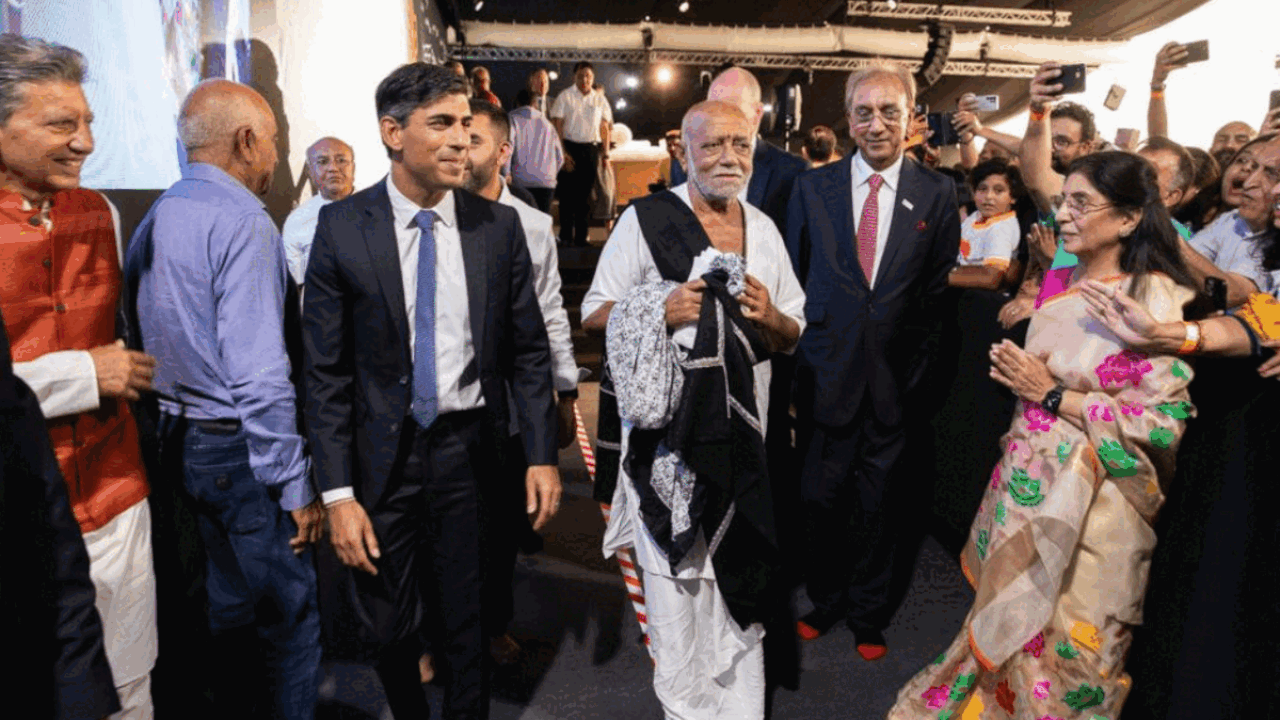The animated GIF consists of three rotating frames, all featuring the British Prime Minister, Rishi Sunak, during what seems to be an official diplomatic visit to India. In the first frame, Sunak is seen smiling and interacting with an audience comprised of people who appear to be Indian, as he walks out of a building. The second frame shows Sunak seated on a cushion, participating in a moment of prayer with an important Indian figure, who is dressed in traditional attire with a black sash across his robe. The final frame captures an audience, including a woman in a floral dress, attentively watching and clapping at his appearance in what seems to be a lecture hall. Sunak’s presence is emblematic of a significant diplomatic event, and he exudes a sense of gratitude and honor throughout the visit, with all participants appearing delighted.